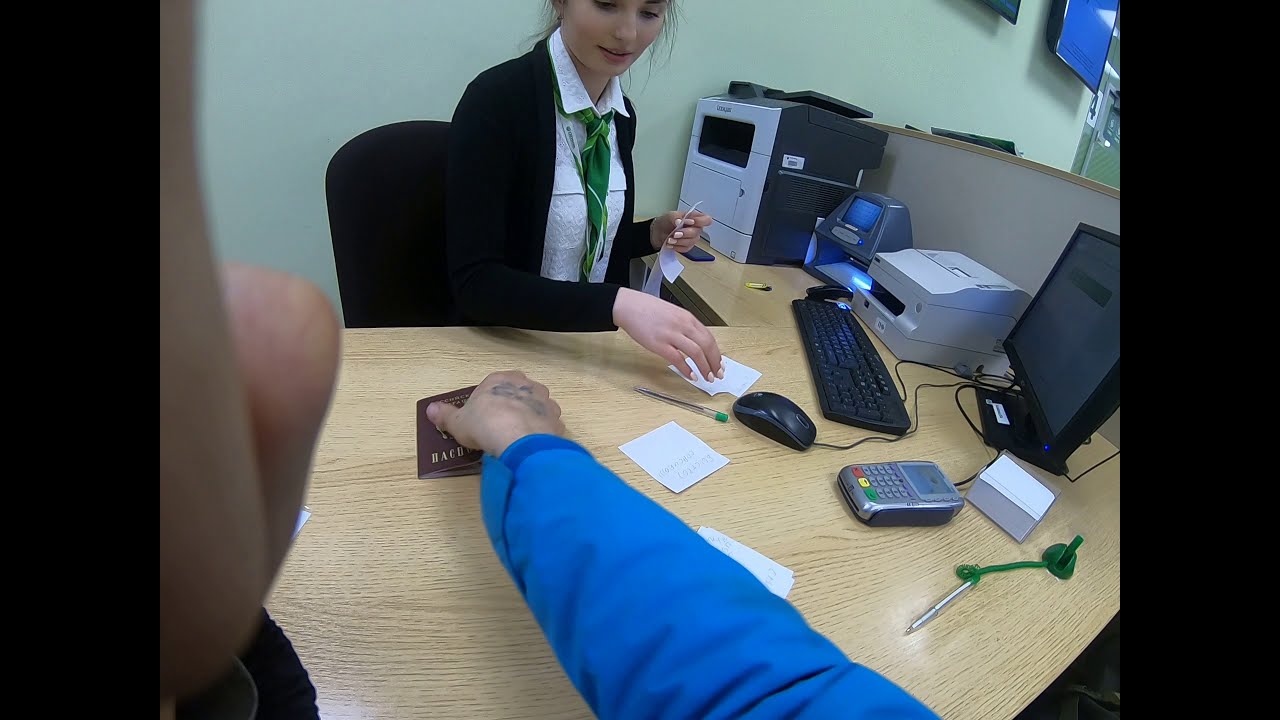In this detailed photograph from an office setting, the perspective is from someone seated at the front of a light brown wooden desk cluttered with various papers and electronics. A person on the left side of the frame, only partially visible, extends their hand to reach for a brown passport with gold lettering. This person wears a long sleeve blue jacket, which contrasts with their darker skin tone adorned with a visible black tattoo. The edge of their face, including the side of their nose and cheek, is barely visible.

The desk is scattered with office essentials, including a silver and black card reader, a black computer monitor, keyboard, and mouse, and various connecting cords. To the right side, a silver pen is tethered to the desk with a green string, next to a stack of white post-it notes. There’s also a black framed computer monitor and a second printer in the corner.

Behind the desk, a woman with pale skin and dark brown, slightly frizzy, pulled-up hair sits in a black office chair. She is dressed in a black cardigan over a white collared shirt paired with a green tie. Her gaze follows the motion of the arm reaching for the passport, her hands poised near her computer mouse and keyboard, ready to input information. This scene captures a typical moment in an office environment, highlighting the interaction between the individuals amidst their surrounding workspace.